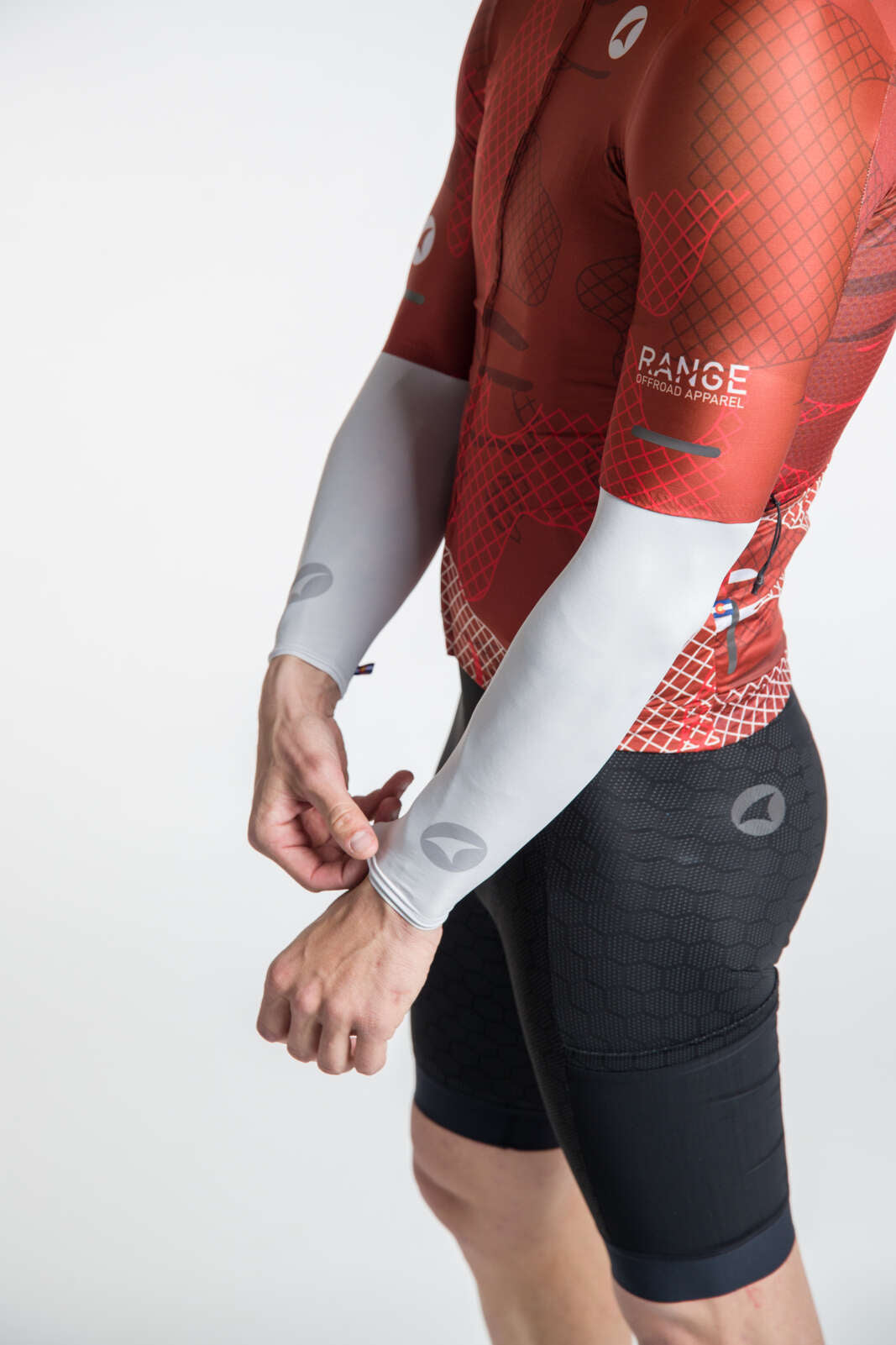This photograph captures the body of an athlete, shown from his shoulders to his knees, with his left side facing the viewer. His pale skin contrasts with his sleek athletic apparel, which includes tight black compression shorts reaching from just above his knees to his hips, featuring a grey honeycomb outline and a darker grey oval logo with a black sail design on the side. He is also clad in a snug, predominantly red shirt adorned with a distinctive pattern: dark red squares on the shoulders, light red squares slightly below, and on the abdomen area. The shirt's white sleeves, which he adjusts with his right hand pulling at the left sleeve, also display an oval silver logo with a white upside-down sail design on the wrist. Additionally, the white oval logo with a red sail is present on his chest and bicep, emphasizing the brand. The text "Range Off-Road Apparel" is imprinted in white on his left arm beneath a red squiggled line. The athlete’s attire and posture suggest readiness for intense physical activity, illustrating the functional and aesthetic design of the Range Off-Road Apparel.